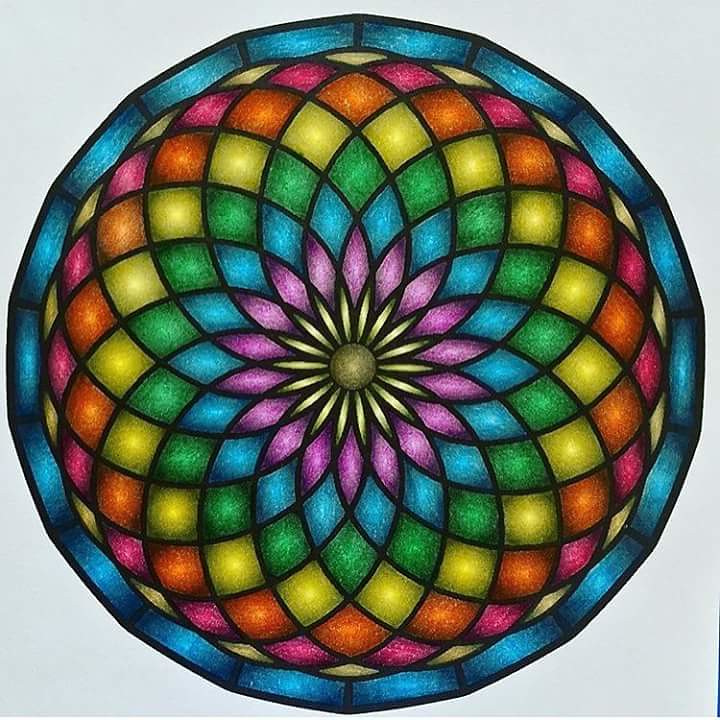Detailed Description:

This is an intricately crafted circular artwork featuring a mesmerizing kaleidoscope pattern. At the heart of the piece lies a brilliant golden flower, which serves as the focal point. Surrounding this central blossom are successive layers of geometrically symmetrical flowers, each expanding in a vibrant array of colors. These layers exhibit a sacred geometry design that resonates outward in perfect symmetry. The progression of colors from the innermost to the outermost layers is as follows: gold, purple, blue, green, yellow, orange, red, and gold. Encircling the entire composition is a final border comprised of blue rectangles, providing a striking frame to this exquisite and harmonious visual feast.